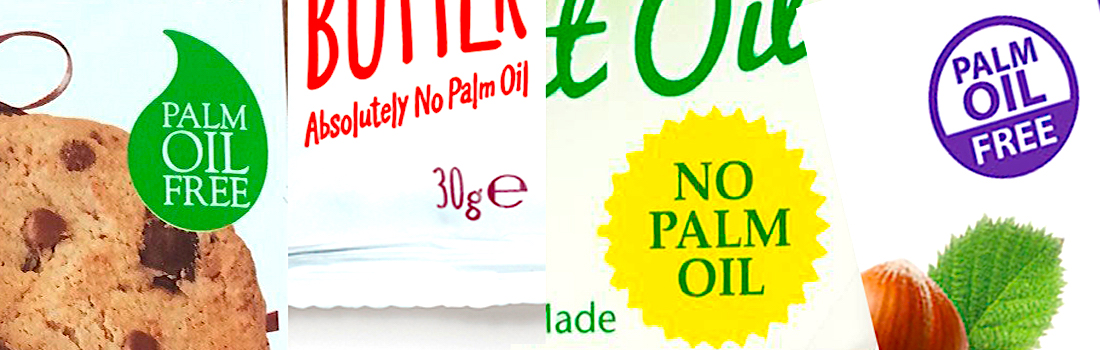The image depicts the front of a box, presumably for a food product such as cookies. Dominating the visual are multiple colorful elements and various texts emphasizing a "palm oil free" message. The left side features a partial image of a chocolate chip cookie layered within a water drop-shaped graphic in green with white text that reads "palm oil free." Adjacent to this, in red text, are the words "absolutely no palm oil," followed by "30g" written in purple. A prominent bright yellow sunburst graphic also reiterates "no palm oil" in green text. Scattered on the surface are motifs of almonds and mint leaves, accompanied by an additional purple circle proclaiming "palm oil free." The boxes are positioned sequentially: the first on the far left, followed closely by the second, third, and fourth. The colors utilized span mint green, light purple, white, yellow, green, burgundy, red, tan, and chocolate brown.